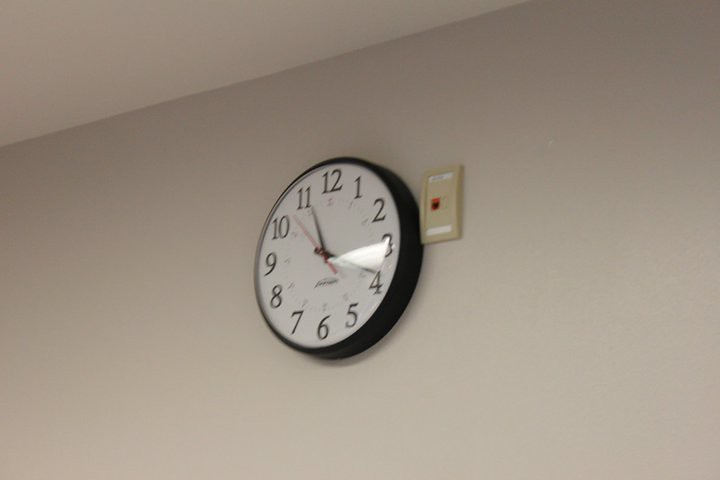In the foreground of the image, there is a prominently displayed clock with a black border. The clock features a white face with black Arabic numerals from 1 to 12, with 12 at the top and 6 at the bottom. Each numeral is accompanied by small ticks marking the minutes and larger lines indicating 5-minute intervals. The clock's hour and minute hands are black, while the second hand is a contrasting red.

Behind the clock, attached to the white wall, there is a faceplate which appears to house an Ethernet or phone jack. The faceplate is tan, and the jack itself is outlined in either dark red or orange. The center part of the jack, where the cable plugs in, is black, and it seems to have a white label with black lettering above it and an empty horizontal space at the bottom.

The wall and ceiling in the background are white, although the lighting in the room casts contrasting shades, creating a nuanced interplay of light and dark across the surfaces.